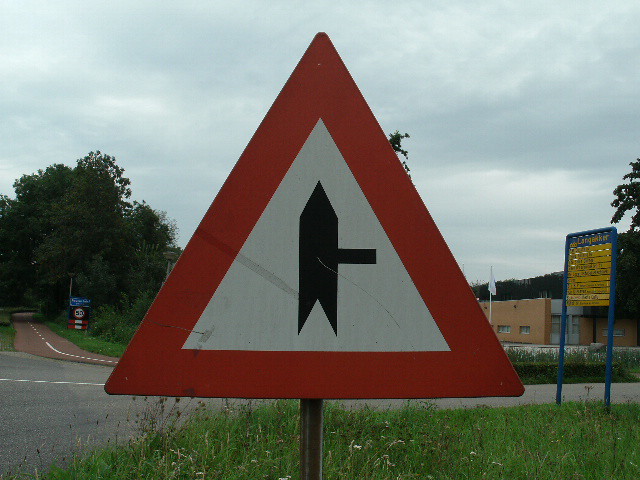This photograph, taken outdoors on an overcast day, captures a scene outside what appears to be an office building or school in a foreign country, as indicated by the unusual street signs. Dominating the center of the image is a triangular sign featuring a red border and a white center with a black, spaceship-like symbol in the middle. The sign lacks text. Surrounding this focal point, the setting includes a grassy field at the bottom right, a small road with a dotted white line, and a parallel sidewalk also marked by white lines. To the left of the triangular sign, the road and walkway stretch into the background. In the back right, there's a speed limit sign and a building with another sign nearby. A white flag flutters against a backdrop of a very gray, cloud-filled sky. The photograph exhibits a palette of red, white, black, green, gray, blue, and yellow, portraying a quiet area with no visible cars or people.